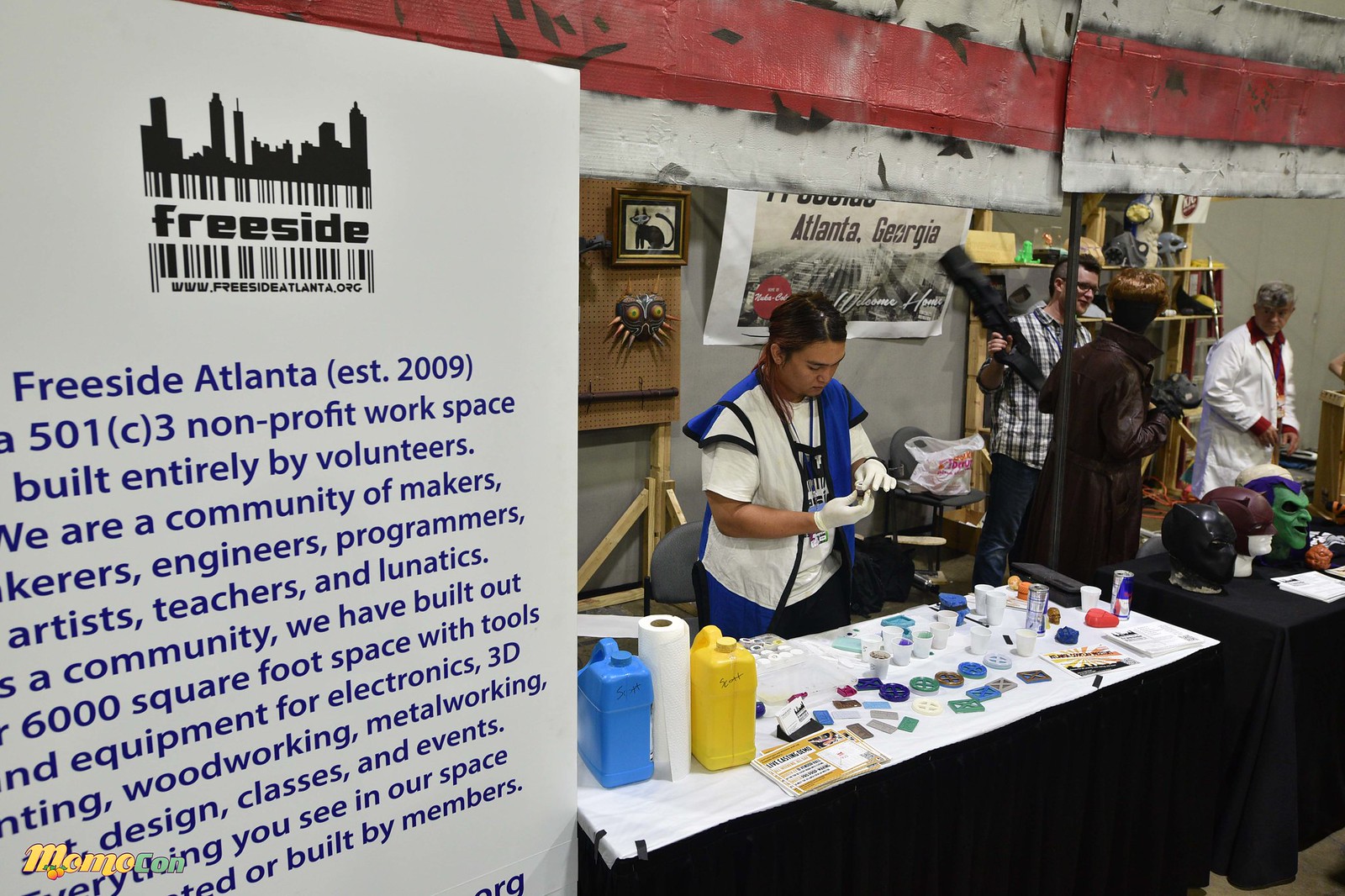The photograph captures an indoor scene of an art event, organized by Freeside Atlanta. On the left side of the image is a prominent white sign with a skyline of black buildings above the bold text "Freeside." The sign reads:

"Freeside Atlanta, Exhibition 2009. Non-profit workspace built entirely by volunteers. We are a community of makers, engineers, programmers, artists, teachers, and lunatics. As a community, we have built our 6,000 square foot space with tools and equipment for electronics, 3D printing, woodworking, metalworking, design, classes, and events. Everything you see in the space is built by members."

In the center of the image, a woman stands behind a display table. She is engaged in mixing colors, possibly to create different colored clays, and the table is cluttered with translucent cups filled with various hues, tools, and two open red bowls. Adjacent to her table, there is another table covered with a black tablecloth, showcasing superhero masks, including Batman and the Joker, as well as an unfamiliar brown mask in the middle.

To the right, there is a man standing at another table with various tools and bottles of liquid, alongside a large blue jug, a roll of paper towels, and a yellow jug. The attendees appear focused on their tasks, contributing to the creative and collaborative atmosphere of the event.